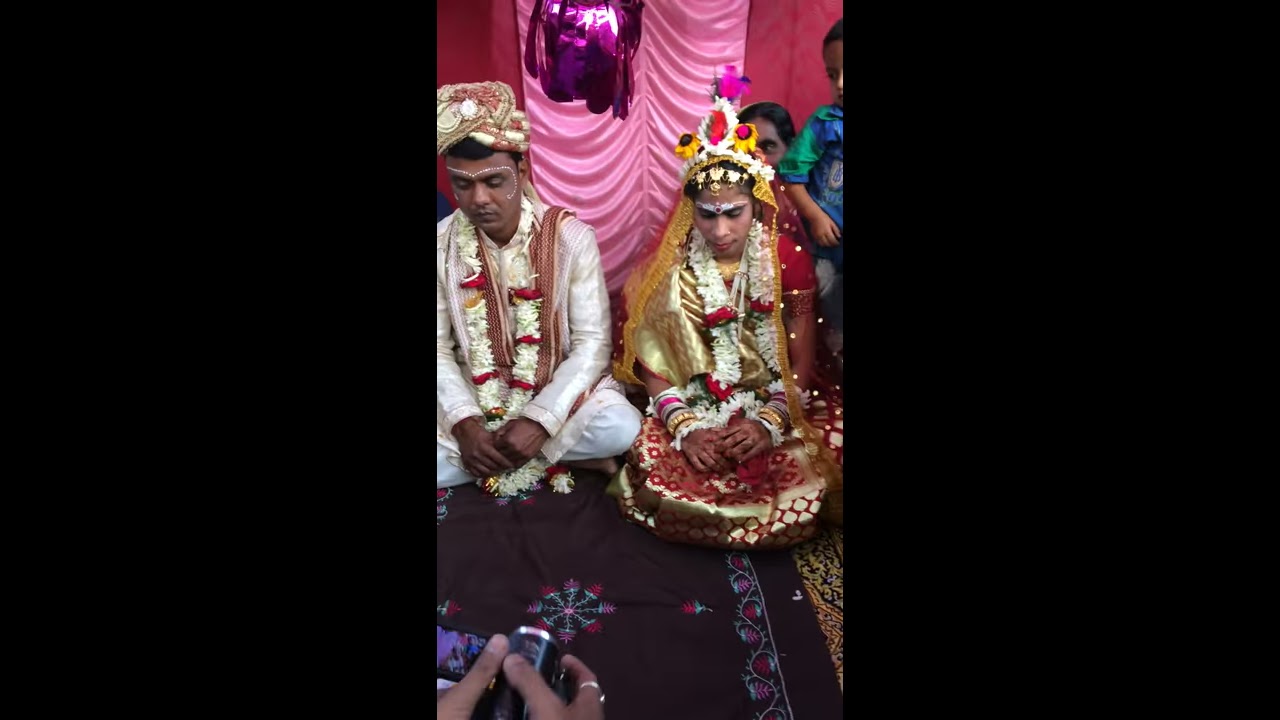This vibrant photograph captures an elaborate Indian wedding celebration set within a pink tent. Seated on a richly decorated brown carpet, the couple is dressed in traditional, ornate attire and are adorned with colorful garlands around their necks. 

The groom, positioned to the viewer's left, is dressed in a pristine white outfit. He wears an elaborate headpiece featuring a blend of white, cream, pink, and brown shades, complemented by a reddish-gold scarf draped over his shoulders. His face is marked with white dots extending across his forehead and cheeks, and his eyes are closed in a serene expression.

Adjacent to him, the bride sits on the right, resplendent in her red and gold gown. Her headdress is particularly intricate, featuring white floral elements with touches of yellow lace-like material hanging from the sides, and gold pieces forming a chain across her forehead. She too has her face adorned with decorative paint and her eyes closed, giving her an equally composed appearance.

Behind the couple, a woman can be seen with a small child in her arms, the child dressed in a blue and green shirt. An obscured individual with dark hair stands further in the background. At the forefront of the image, a black material-like blanket is partially visible, with a pair of hands holding a black object, rings adorning the fingers.

This image captures the essence of a deeply traditional Indian wedding, replete with rich colors, intricate decorations, and a sense of solemnity around the couple, who appear deeply immersed in their ceremonial moment.